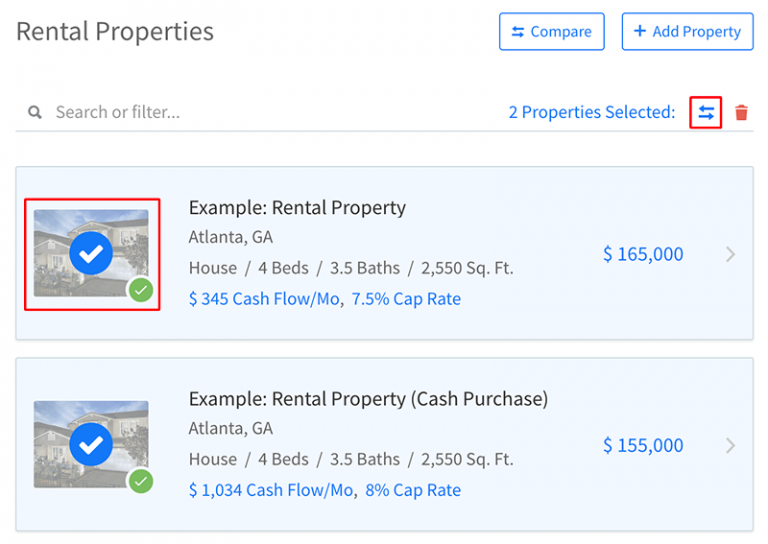The image displays a mostly white background with a subtle hint of light blue. The focal point of the image features two boxes each containing specific information. 

Above these boxes, there's a single bar with some text. To the left, you see the phrase "Rental Properties," while on the right there are two buttons with blue text that read "Compare" and "Add Properties." Below these buttons, there is a magnifying glass icon followed by the words "Search" or "Filter," followed by three dots. Next to this, it shows "2 properties selected," accompanied by a red square containing stacked arrows pointing left and right. Adjacent to these arrows is a red trash can icon.

In the first box, there is a large house image bordered by a red square. Superimposed on the house are a blue checkmark covering the front of the house and a green checkmark at the bottom corner near the front lawn. Below this image, the text describes the property as "Example Rental Property, Atlanta, Georgia." Details include:
- Type: House
- Bedrooms: 4 
- Bathrooms: 3.5 
- Area: 2,550 sq ft
- Cash Flow: $345 per month
- Cap Rate: 7.5%
- Price: $165,000

The second box is similar, with another image of the same house, but without the red border. It also features the same blue and green checkmarks. However, the description text differs slightly, reading "Example Rental Property, Cash Purchase, Atlanta, Georgia." Details include:
- Type: House
- Bedrooms: 4 
- Bathrooms: 3.5 
- Area: 2,550 sq ft
- Cash Flow: $1,034 per month
- Cap Rate: 8%
- Price: $155,000